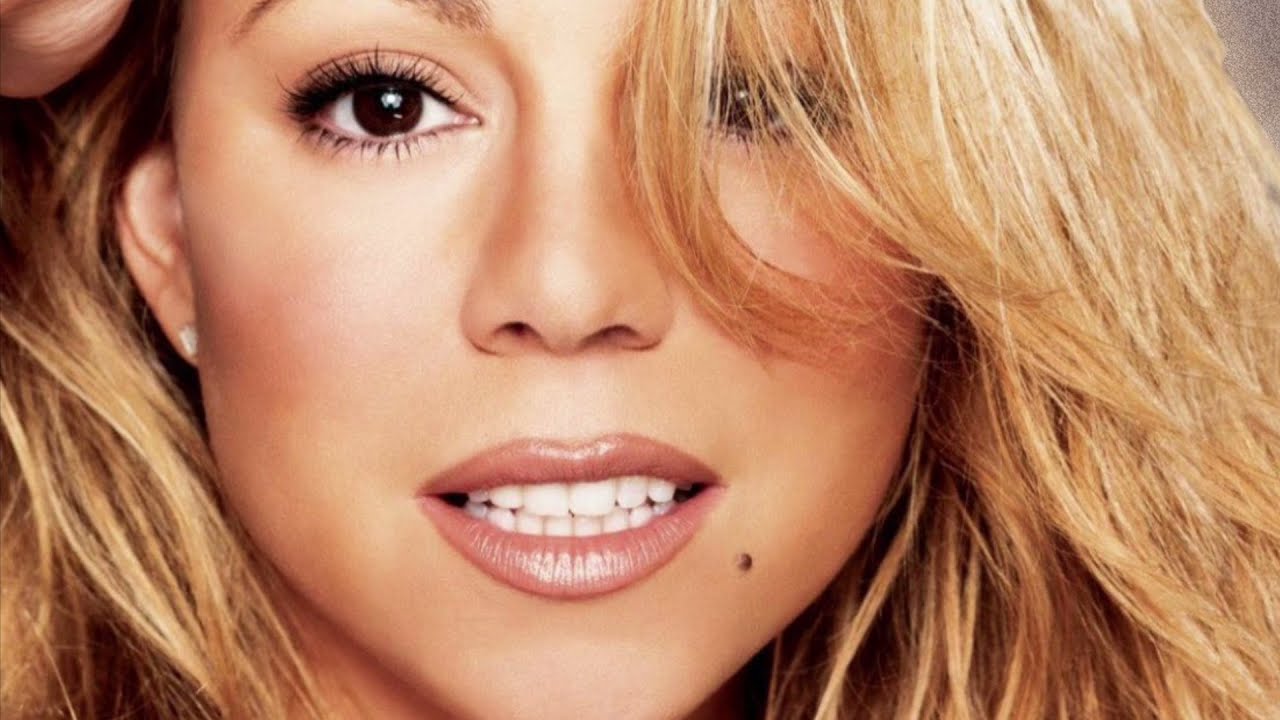This close-up photograph, likely of Mariah Carey, captures an intimate and detailed view of her facial features. The rectangular image, with dimensions similar to a high-definition television screen, frames her from the eyebrows to the chin. Mariah's light brown to blonde hair cascades over the right side of her face, partially obscuring her right eye. Her large, glossy brown eyes exude warmth, while her perfectly white teeth are visible behind her slightly open, pink lips. A distinct black mole punctuates the right side of her lower lip on her cheek. She wears minimal yet distinct makeup, with pinkish lipstick and noticeable reddish blush on her cheeks. Both her upper and lower eyelashes are enhanced with mascara, and a hint of eye shadow complements the look. A diamond or clear stud earring adorns her left ear, partially hidden by her hair. In the top left corner of the image, a subtle part of her hand is visible, as if she is holding back her hair. No background details are evident, emphasizing the close-up nature of this evocative portrait.